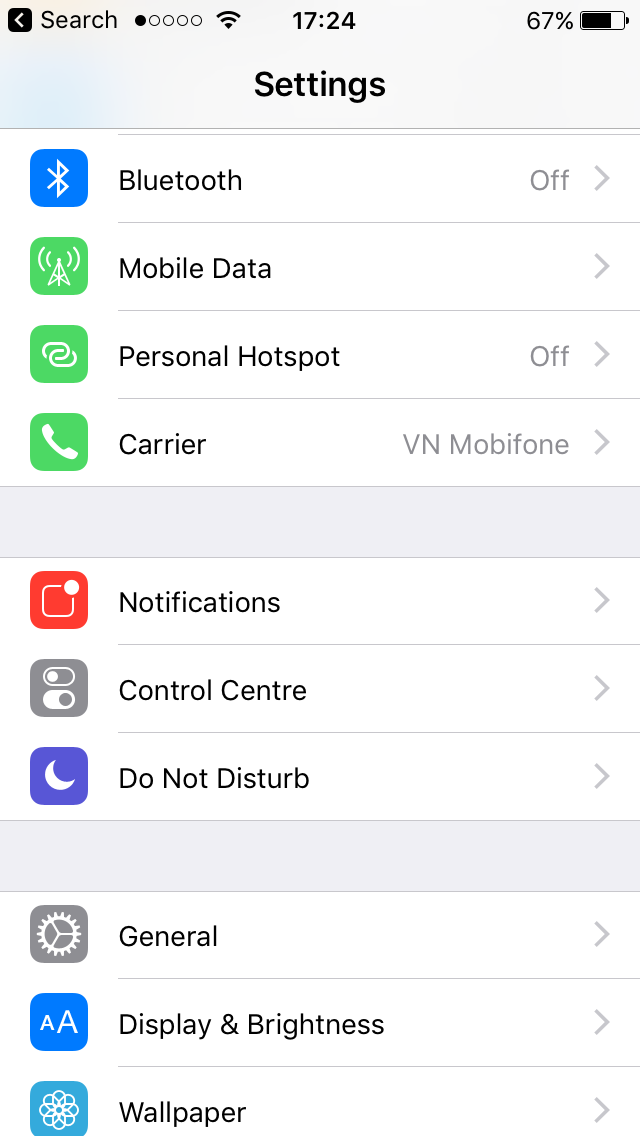An image showing the screen of a smartphone displays various settings menus. At the top of the screen, there is a back button labeled "Search." Below this, five small circles are displayed, with only one filled in black while the remaining four are white. Directly below, a swirling icon indicating connectivity is visible next to the time, which reads 17:24. To the right, the battery level is indicated at 67%, with a partially filled black bar representing the remaining charge.

The screen is divided into three sections: top, middle, and bottom. In the top section, there are settings options for Bluetooth, Mobile Data, Personal Hotspot, and Carrier, each accompanied by an icon. The Bluetooth icon is within a blue box, while the remaining icons are within green boxes.

The middle section follows, separated by a gray horizontal rectangle. This section includes settings for Notifications, Control Center, and Do Not Disturb. Further down, separated by another gray horizontal rectangle, the bottom section includes settings for General, Display & Brightness, and Wallpaper. Each option is paired with its corresponding icon and a right-pointing arrow, indicating further settings or sub-menus are available for each option.